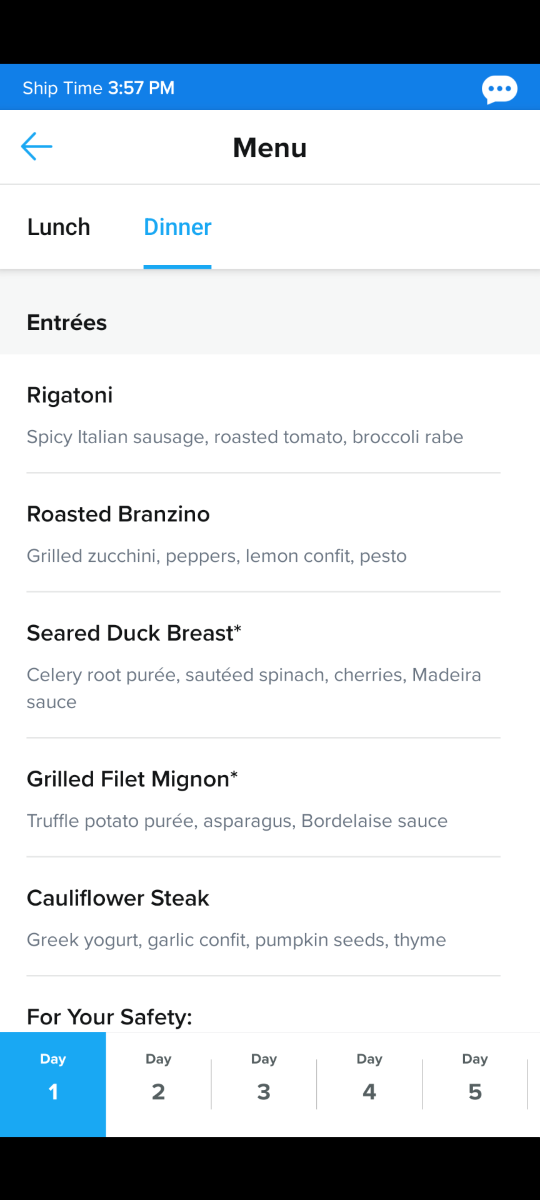The mobile phone screen displays a menu interface. At the very top is a black rectangular bar, followed by a smaller royal blue bar that reads "Ship Time 3:57 p.m." in white text, accompanied by a white speech bubble with three dots inside it. Below this, the background transitions to gray with a faint gray line separating each section of the user interface.

The screen prominently features a blue left-pointing arrow labeled "Menu." The menu is divided into sections for "Lunch" and "Dinner," with the "Dinner" section highlighted in blue and underlined, indicating it is currently being viewed. Under the "Entrées" category, listed against a gray backdrop, are the following items:

1. **Rigatoni** - Spicy Italian sausage, roasted tomato, broccoli rabe.
2. **Roasted Branzino** - Grilled zucchini, peppers, lemon confit, pesto.
3. **Seared Duck Breast*** - Celery root puree, sautéed spinach, cherries, Madeira sauce.
4. **Grilled Filet Mignon*** - Truffle potato puree, asparagus, bordelaise sauce.
5. **Cauliflower Steak** - Greek yogurt, garlic confit, pumpkin seeds, thyme.

Each entrée is separated by a faint gray line. The section ends with a note labeled "For your safety:" followed by additional text not fully visible. 

Below this, the menu features a series of five boxes representing different days. The first box, highlighted in blue with white text, reads "Day One," indicating the current selection. The subsequent boxes, in white with black text, read "Day Two," "Day Three," "Day Four," and "Day Five," separated by vertical lines. 

At the bottom of the screen, there is another black rectangular bar.